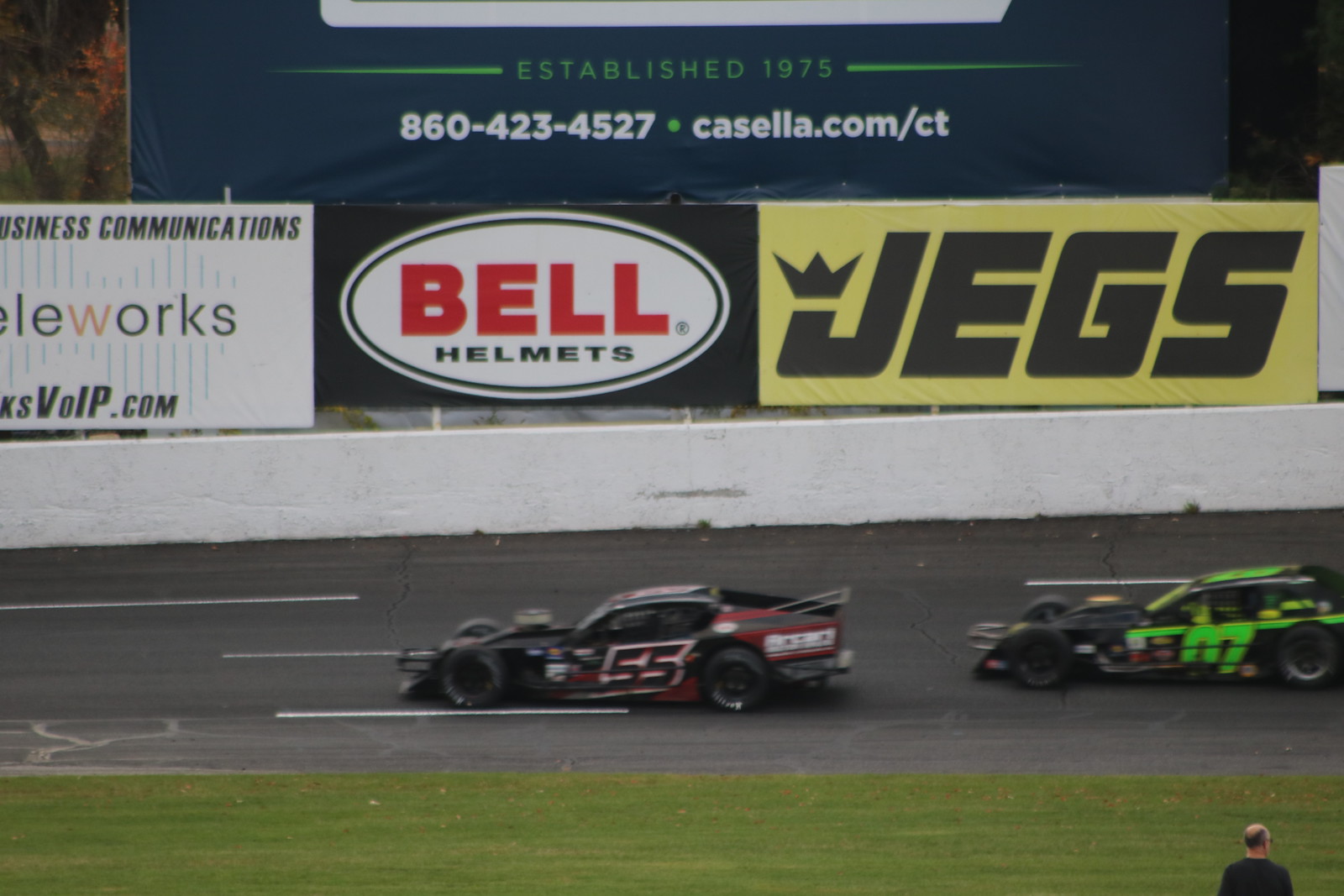The image captures a vibrant and detailed scene at a racetrack. In the foreground, there is a grassy section just before the track, where a man, visible from the shoulders up, is standing in the bottom right corner; he appears to have gray hair and is wearing a dark t-shirt. The race track itself is made of black asphalt with white lane markers, and two cars are speeding from right to left. The lead car is numbered 55, featuring a black, red, and white color scheme, while the trailing car is black with green graphics and possibly the number 07. Both cars are in motion. Behind the track, there is a white half-wall adorned with various sponsor banners. These include a white sign partially visible with the words "communications works," a black banner with a white oval and red text reading "Bell Helmets," and a yellow banner reading "JEGS" in bold black capital letters with a crown over the "J." Another sponsor mentioned is Casella, referencing Connecticut roots. The photographic style is highly detailed, emphasizing realism and representationalism.